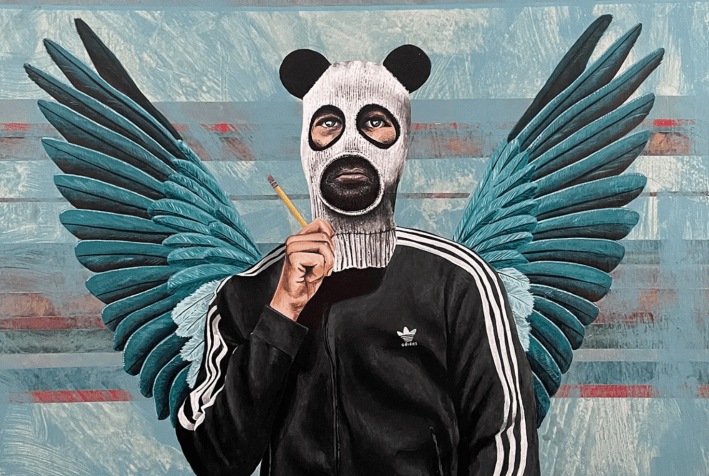The image showcases a man posing in front of a mural comprised of red, white, green, and black stripes painted on a building. The mural’s style evokes the aesthetic of a tattoo or graffiti artist. The man, who has a bearded face partially covered by a knit cap with panda bear ears, wears a black Adidas track jacket adorned with white stripes on the sleeves and the Adidas logo on the left chest. The backdrop behind him cleverly incorporates large, vivid blue wings, giving the illusion that the man has these wings sprouting from his back. He's holding a No. 2 pencil in his hand, and his eyes and mouth are visible, suggesting that the face mask or ski mask he wears does not obscure them. The background also features hints of blue shading and possibly some railing with red, gray, and blue accents, further enriching the scene.